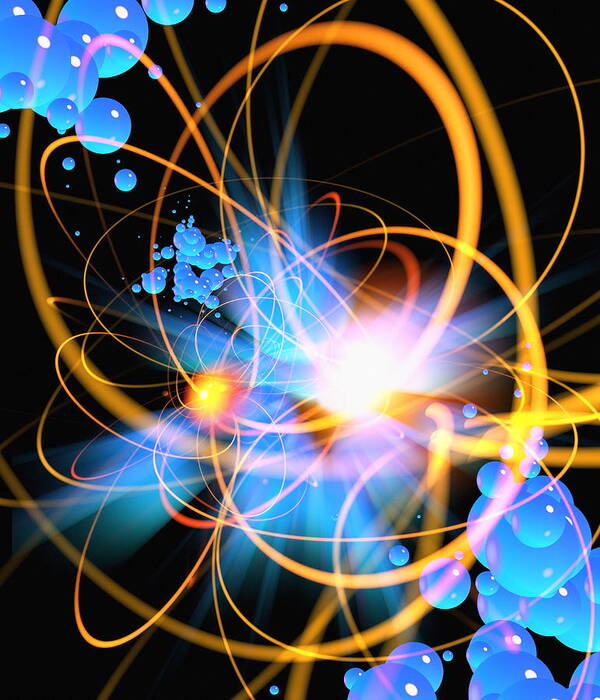This abstract, science-themed animated illustration features a dramatic solid black background, punctuated by vibrant visual elements. Dominating the center, a large, bright whitish-yellow light reflects outward, giving the impression of a neutron-like entity. From this focal point, numerous golden, curly lines loop outward in all directions, reminiscent of light path photography's glowing effect. Surrounding this central light, ethereal blue rays emanate, creating a striking contrast against the dark backdrop. Additionally, clusters of bubbles in varying shades of blue, green, purple, and white are scattered across the composition, primarily concentrated in the top left and bottom right corners, adding dynamic movement throughout the rectangular portrait view.